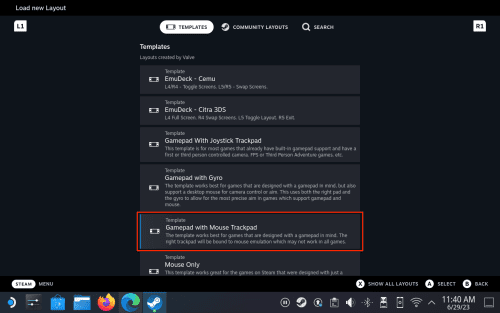The image displayed on a computer screen is horizontal and rectangular. The top section of the screen is a dark black bar, featuring the text "Load New Layout" in white font positioned in the upper left-hand corner. Directly below this is a slightly lighter black section that occupies the majority of the screen. 

In the upper left area of the lighter black section, there is an icon. Dominating the center of this section are three main elements: a white oval with the word "TEMPLATES" written in bold, black, capital letters accompanied by an icon on the left, a black rectangular area with the text "Community Layouts" in white font and another icon to its left, and a search bar labeled "Search," also with a magnifying glass icon to its left.

Below this central area, the screen displays a list of horizontal rectangular sections in an even lighter black hue, each separated by thin, black dividing lines. There are six of these rectangles, and their text is quite small and difficult to read. Each appears to have some form of abbreviated or coded name such as "E-M-DEC-C-E-M-U." Notably, the fifth rectangle is outlined with a red border and is legible, displaying the text "Gamepad with Mouse Trackpad."

At the bottom of the screen, a very dark border runs the width of the image, containing various words. The lowest part of this border partially cuts off the final rectangular section of the list. The very bottom edge of the image features several icons representing different web browsers and the current time displayed in the right-hand corner.